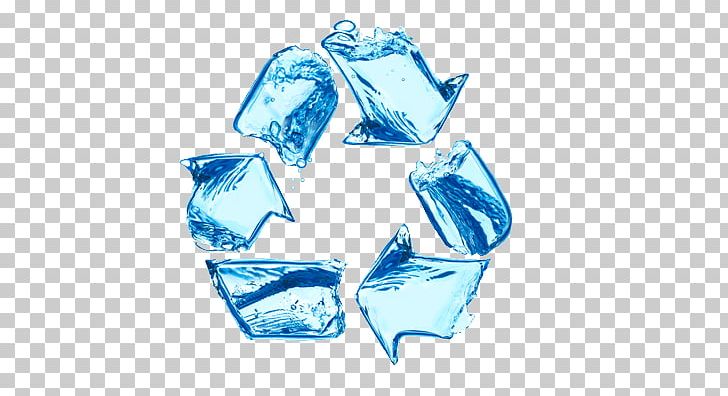The image features a wide horizontal rectangle with a gray and white checkerboard pattern as the background. The checkerboard is composed of evenly distributed small squares. Centrally positioned is a blue recycling symbol, characteristically shaped as a triangular loop made up of three arrows. Each arrow transitions fluidly into the next, forming a cohesive triangular pattern. The arrows are artistically designed to resemble water, with light blue hues mingled with darker blue accents and visual elements suggesting bubbles or waves. There are no additional objects or text present in the image, ensuring the focus remains solely on the water-inspired recycling symbol against the simple checkered backdrop.